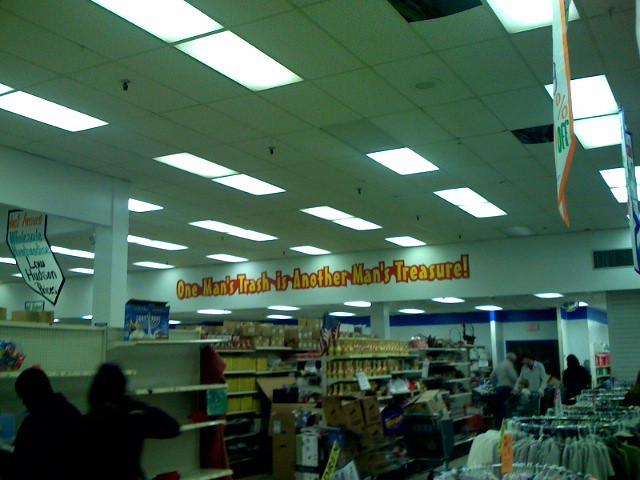The image captures the interior of a department store, albeit in a blurry and low-resolution photograph. High ceilings adorned with commercial-style tiles and illuminated by fluorescent lighting dominate the scene. On the far wall, a white surface bears the phrase "One man's trash is another man's treasure" written in a prominent yellow font. Below this motivational slogan, several aisles filled with various goods can be faintly discerned, although the details are obscured due to the photo's blurriness. Piles of boxes are scattered in the middle of the store, adding to the sense of clutter. To the right, racks brimming with clothes are visible, contributing to the overall sense of organized chaos. The presence of a few indistinct, blurry figures suggests that shoppers are navigating this space. Despite the lack of clarity, the image conveys a bustling, somewhat haphazard retail environment.